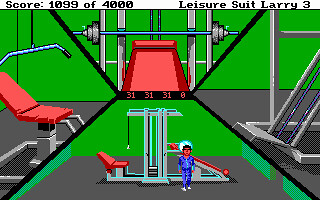The image captures a video game screen featuring "Leisure Suit Larry 3." At the top of the screen, the player's score is displayed: "Score: 1099 of 4,000." The scene is set in a gym, showcasing various workout equipment. Prominently featured is a bench press with a red backrest, marked with the numbers "31 31 31 0." Above the bench is a barbell for performing presses.

To the left, a shoulder press machine is visible, equipped with a red chair for back support and a long, angled bar designed to be pulled down. On the right, there's an unidentified piece of equipment with two gray columns and matching gray supports, though its specific function isn't clear.

The entire gym setup, comprising a gray-framed total gym system, occupies the bottom section of the screen. In the center of this system, a stack of weights is prominently displayed, which move up and down with the shoulder press machine. In the foreground stands the character Leisure Suit Larry, clad in his signature blue leisure suit, positioned in front of this comprehensive gym setup.